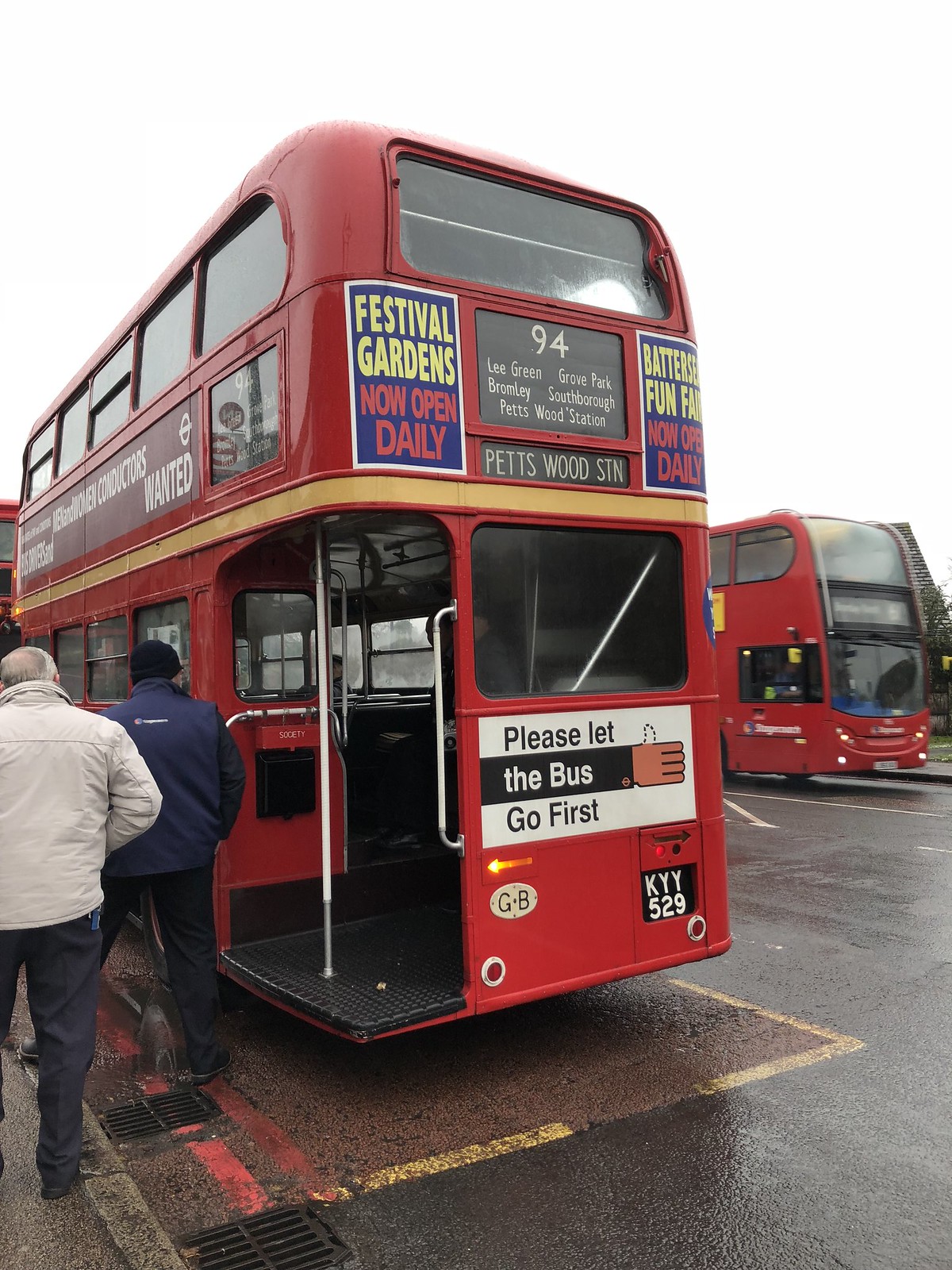The photograph captures a bustling outdoor scene at a bus station during daytime. Dominating the center of the image is a red double-decker bus adorned with various advertisements and signs. One prominent sign reads "Festival Gardens, now open daily" and another says "Please let the bus go first." The bus is identified as route number 94, headed to Petswood station, with the station name intriguingly spelled as "Pettswood." The license plate visible on the bus is "KYY 529."

Toward the middle left of the image stand two men poised to board the bus. One man wears a beige jacket and dark pants, while the other sports a blue jacket with dark pants and a cap. The pavement underfoot appears wet, and several drainage vents are noticeable on the ground. The backdrop reveals another red double-decker bus, which seems slightly more modern. The sky overhead is a glaring white, contributing to the overall bright daytime ambiance. The setting, enhanced by the various colors such as black, yellow, red, orange, blue, gray, maroon, and white, clearly indicates it is a busy moment at the station.